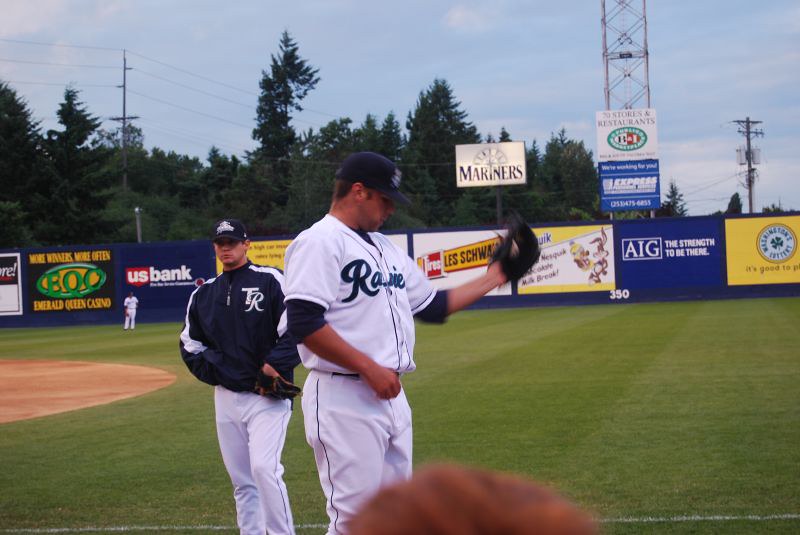This bright and clear horizontal rectangular photograph captures a moment on a baseball field. Centrally positioned, a baseball player in a white uniform with text across his chest stands with a black glove on his left hand, appearing to hold a ball. Behind him, another player, slightly further away, dons a dark blue jacket emblazoned with the initials "TR" over white trousers and a dark blue cap. A third player in the background also wears a white jersey and trousers, along with a dark blue cap, standing close to the park's high, dark blue wall which features multiple advertisements including those for AIG, US Bank, Mariners, and Express. The lush green grass of the infield extends to the wall lined with billboard signs. In the distance, dense green trees and a radio tower are visible under a lightly clouded blue sky, along with telephone poles on the far right.